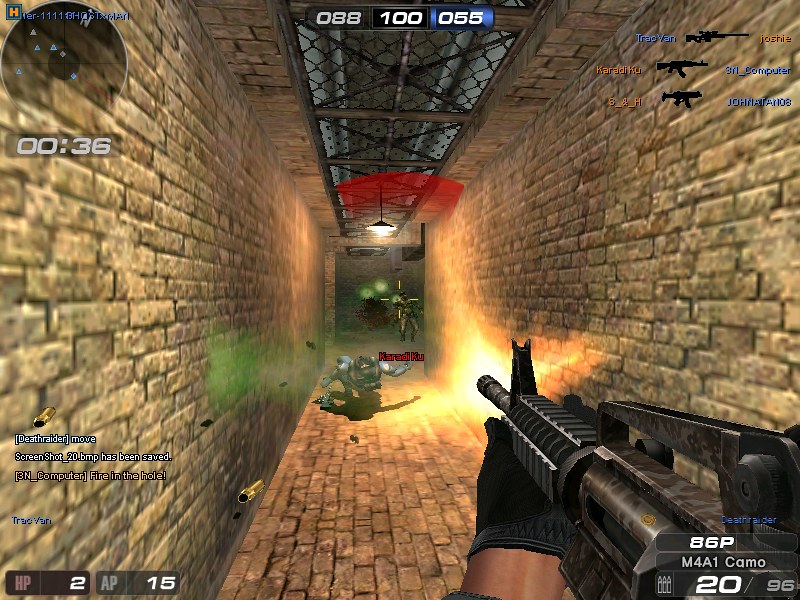A screenshot from a first-person shooter video game showcases intense combat action. In the image, the player's character is holding a rifle in their right hand, actively firing at enemy combatants. The scene takes place in a gritty, brick-walled tunnel, featuring a mesh grate on the ceiling that adds to the underground, industrial atmosphere. Various game icons are subtly displayed around the edges of the screen, providing additional gameplay information. At the top of the image, three numerical indicators read 0 8 8, 100, and 0 5 5 respectively, with a countdown timer showing 36 seconds remaining, adding a sense of urgency to the scenario.